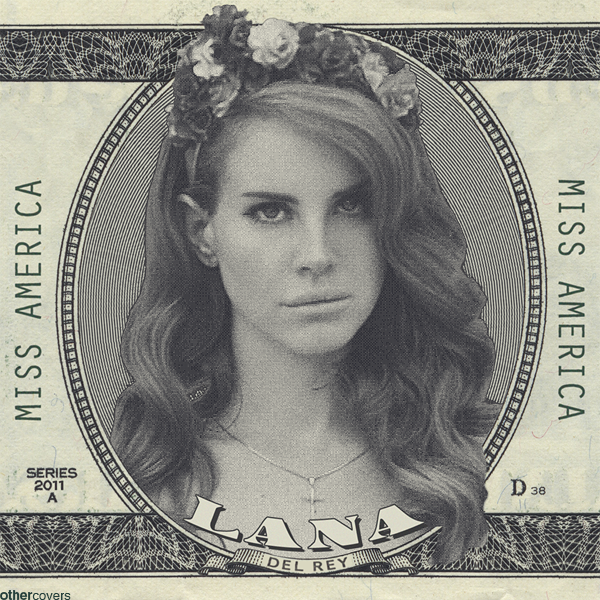The image is a meticulously photoshopped montage of Lana Del Rey featured inside a dollar bill's portrait, replacing George Washington. The design adopts the motif and style of U.S. currency, predominantly presented in black, white, and light green hues. Lana Del Rey, shown from the chest upwards, gazes directly at the camera with long flowing hair adorned with a flower garland. She wears a necklace with a pendant shaped like a cross. The portrait is framed within the intricate oval typical of a dollar bill. The left and right sides of the image declare "Miss America" in capital letters. At the bottom, rendered in a formal typeface, it reads "Lana Del Rey." Additionally, details such as "Series 2011A" appear at the bottom center, while "D38" is noted at the very bottom right. The lower left corner mentions "other covers", indicating additional montage or thematic elements.